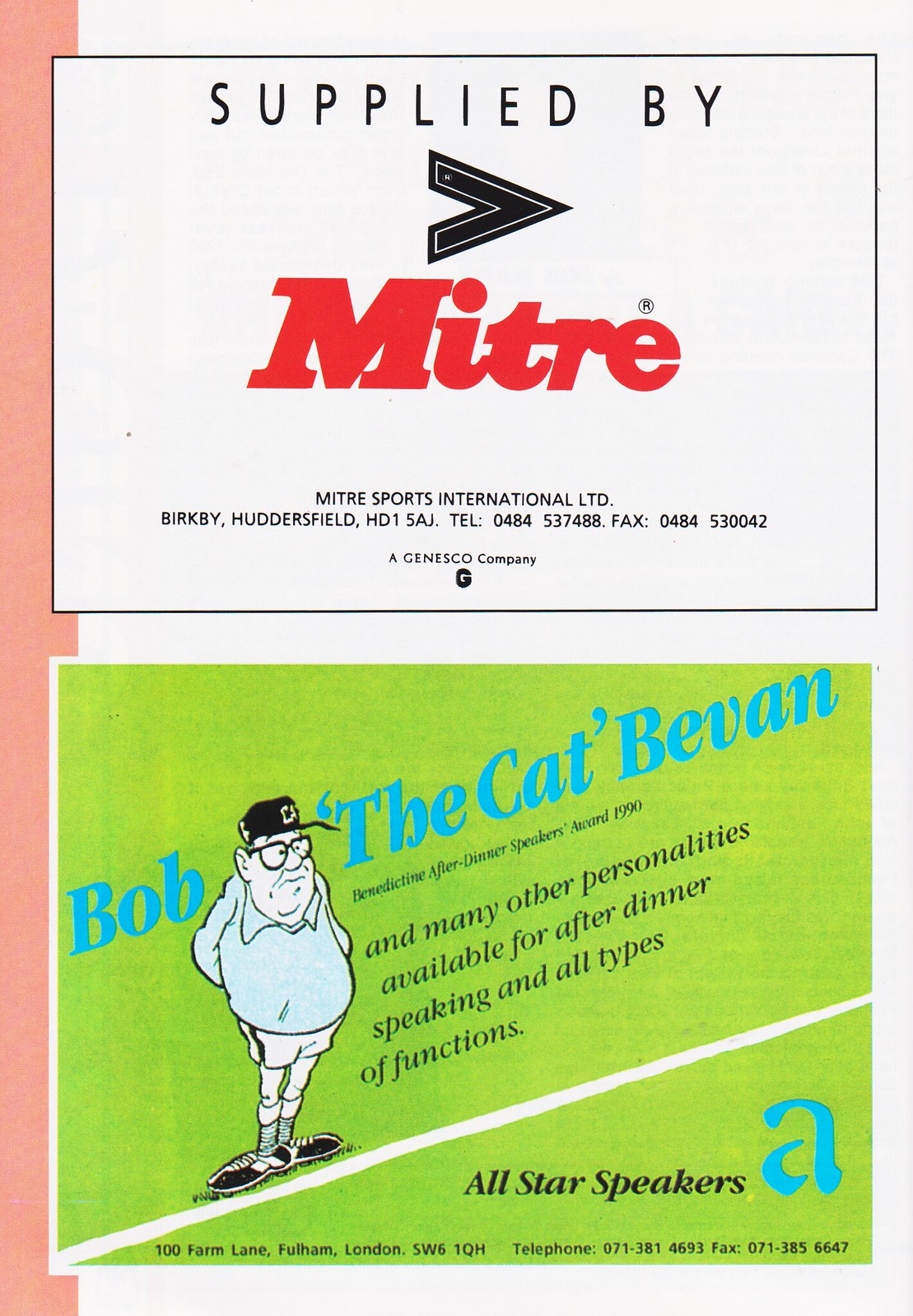The cover image of this sports program or advertisement is in portrait orientation and divided into two distinct halves. The top half features a white square with a black border and includes a bold red italic headline reading "MITRE," preceded by the words "Supplied by" with a right arrow symbol. Below this, the text reads "MITRE Sports International Limited" along with the address "Burt B. Huddersfield HD1 5 AJ." It also provides a telephone number "0484 537 488" and a fax number "0484 530 042," followed by the notation "A Ginesco Company."

The bottom half of the page shows a lime-green square resembling a baseball field. Dominating this section is a line art illustration of a cartoon man wearing a black ball cap, a polo shirt, shorts, and sneakers. The man stands above a line with the blue text "Bob 'The Cat' Bevan" prominently displayed near him. Additional text mentions his availability for after-dinner speaking and various functions. The bottom right corner contains a logo and text for "All-Star Speakers," including the address "100 Farmland, Fulham, London SW6 1QH," along with the telephone number "071 381 4693" and fax number "071 385 6647."